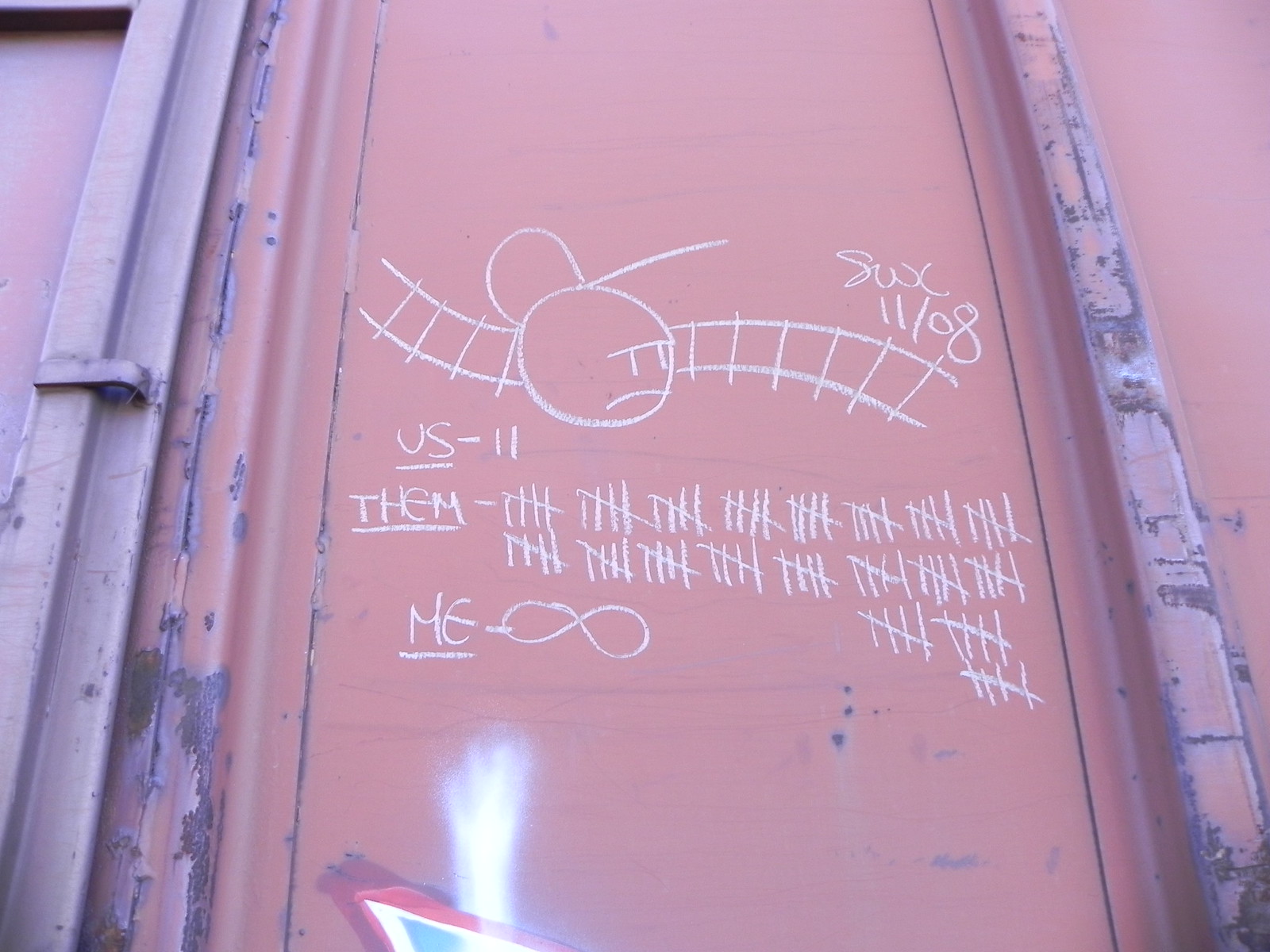The image displays a close-up of a pinkish-brown metal industrial-style door, embedded into a matching wall with visibly chipped paint revealing the metal underneath. A rusted pipe runs vertically along the left side, secured to the wall with brackets. Scrawled in white chalk on the door is a detailed graffiti drawing: a wavy railway track with a circular head featuring sad facial expressions—eyes represented by vertical lines and a downturned mouth. Above the drawing is the inscription "11/08" and "US-11," while beneath it, "them" is depicted with tallies indicating a score, each tally consisting of four vertical lines crossed by a diagonal line, suggesting a count of approximately one hundred. Additionally, the word "SUX" appears chalked in the top right corner, and there’s a symbol resembling an infinity sign beneath the tally marks. The drawing and markings suggest someone's attempt to keep score of an unknown game or event.